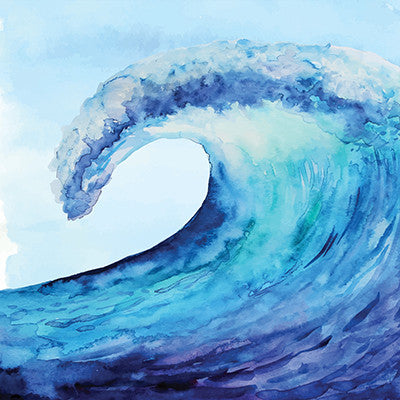This image showcases a stunning painting of a single wave in the ocean, captured in exquisite detail. At the base, the wave is rendered in deep, moody hues of blackish-gray and the darkest blues. Broad, diagonal strokes sweep from the lower left to the upper right, culminating in the crest of the wave. Here, the artist skillfully integrates more white, highlighting the wave as it arches dramatically. As the wave curls backwards, the color transitions to predominantly white with hints of light blue, emphasizing the frothy foam at the peak. The painting conveys a palpable sense of movement, with the artist's energetic strokes vividly depicting the rapid, surging motion of the water. The background features a serene sky in the upper left, painted in soft shades of light blue and white, without distinct cloud formations, creating a harmonious contrast with the dynamic, crashing wave.